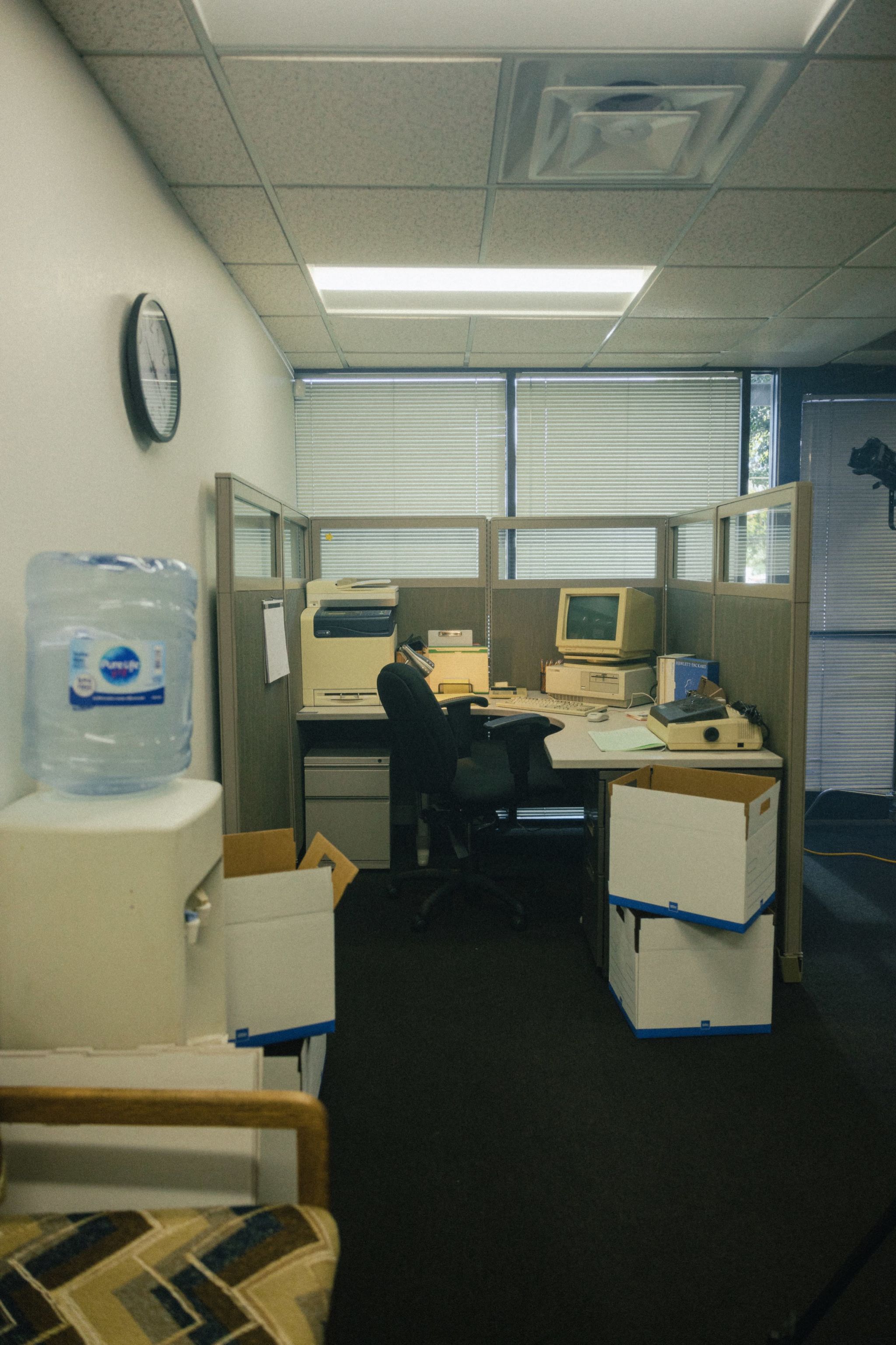The photograph features a scene from an indoor office, possibly reminiscent of the mid-80s to early 90s setup. Central to the image is a cubicle with a small desk. Dominating the desk is an old boxy early nineties-style computer, with a thick CRT monitor perched on a horizontally laid tower, both having aged to a graying yellow hue. Adjacent to the computer on the left rests a similarly antiquated graying yellow copy machine. The office space is enclosed with three-quarters high gray cubicle walls and, behind the desk, windows with drawn blinds that obscure any outside view.

To the left of the main desk area stands a beige water cooler with a water jug upside down, ready for dispensing water, placed near a partial view of a chair and some scattered empty boxes. Close to this setup, on the wall, hangs a round clock. The ceiling above consists of an industrial drop ceiling with square tiles, an air conditioning or heating duct, and fluorescent lights providing illumination.

A corner desk is visible within the cubicle, accompanied by a black office chair upfront and a filing cabinet tucked underneath on the left. Atop this cabinet lies a dated printer. On the desk surface, in front of the monitor, we spot a keyboard and a mouse, with some manila folders arranged in a file holder nearby. Various boxes are scattered around, indicative of ongoing organization or storage. Completing the office aesthetic is a standard blue industrial carpet covering the floor.